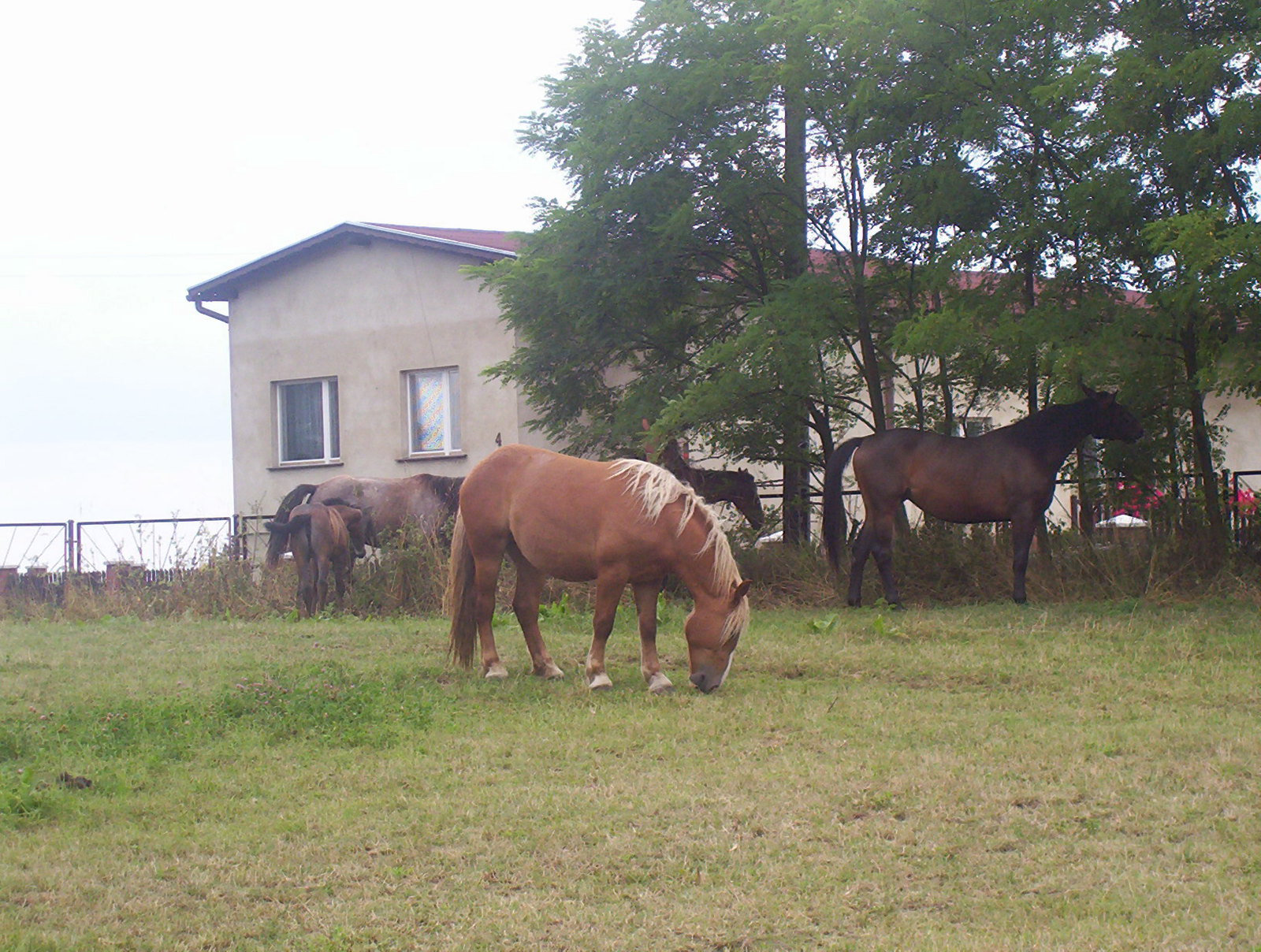In this photograph, taken during an overcast daytime, we see a tranquil backyard scene with numerous interconnected rectangular gray fences lining the perimeter. The fences are adorned with plants that are beginning to brown due to seasonal changes, interspersed with lighter green foliage. Towering trees with dark green leaves cascade over parts of the fence, providing shelter over the horses grazing nearby.

Central to the image are five horses set back in a light green grassy field, speckled with patches of brown and bare mud. The prominent horse in the foreground is a striking golden brown with a light-colored mane and tail, its head bent down as it grazes. Behind it, partially hidden, is a dark brown horse, almost black around its head, neck, and legs. Further in the background, three additional horses are visible with varying shades of dark brown coats.

Beyond the field, a tan house with beige discoloration just below the red roof is visible. This one-story concrete house features two large windows on its left side, each adorned with round banisters - one window having black curtains, the other white. The overcast sky above presents a grayish-blue hue, blending with the white-out effect caused by the brightness levels, rendering the sky nearly white.